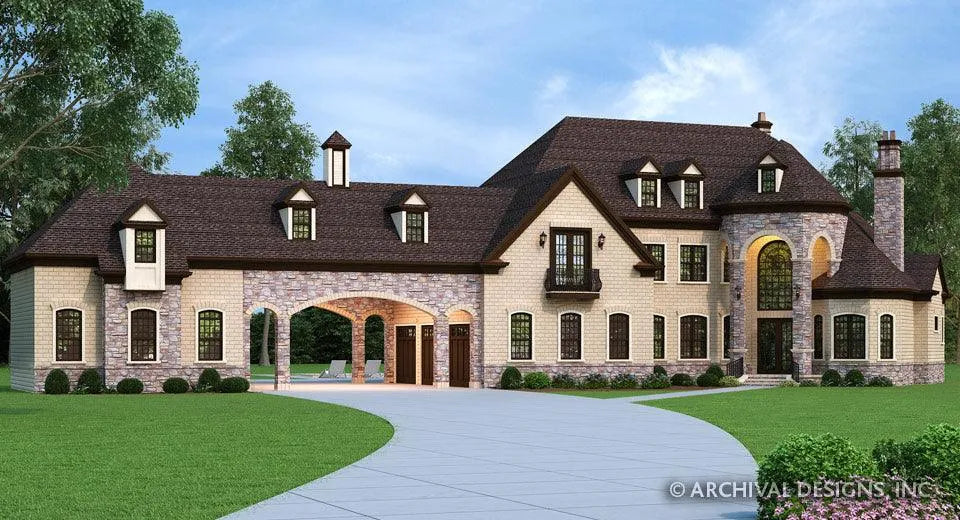This detailed illustration presents a digital rendering of a luxurious, Tudor-style home, showcasing the architectural plans designed by Archival Designs Incorporated, as indicated by the copyright in the bottom right corner. The house, crafted from yellow stone and cream brick, features a dark brown tile roof and numerous arches, including a striking U-shaped cobblestone archway to the right. The central curved driveway guides to a covered carport section, framed by a stone archway with a brown roof, which provides access to the main house through three doors. This main structure boasts large brown windows, including a prominent window with a balcony, and multiple dormer windows that add to its intricate design. A secondary structure, possibly a storage area or a mother-in-law suite, is positioned to the left. The meticulously landscaped grounds highlight a well-manicured lawn adorned with trees, bushes with pink flowers, and a clear blue sky with scattered clouds, creating a harmonious blend of nature and refined architectural elegance.